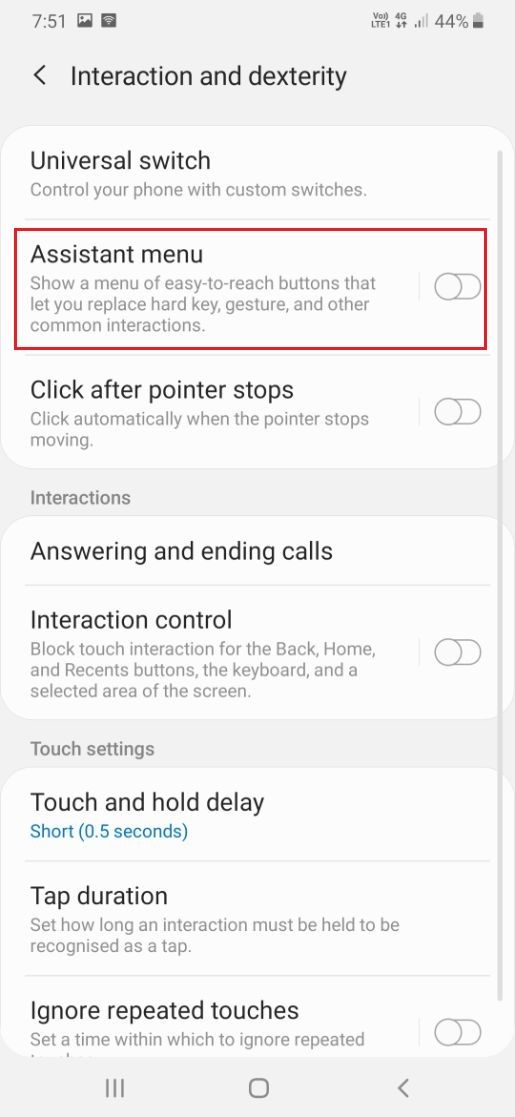This screenshot, taken from a cell phone at 7:51, displays various status icons at the top of the screen, including a screenshot icon, Wi-Fi icon, LED icon, 4G icon, cell reception graph, and a battery icon indicating 44% charge. The main heading reads "Interaction and Dexterity," featuring a back arrow icon. Beneath this, a description of the "Universal Switch" feature mentions its function: "Control your phone with custom switches." Highlighted in a red-lined box is the "Assistant Menu" option, described as "Show a menu of easy-to-reach buttons that let you replace hard key gestures and other common interactions," which is currently checked off, indicating it is inactive. Below this, another inactive option, "Click after pointer stops," is shown.